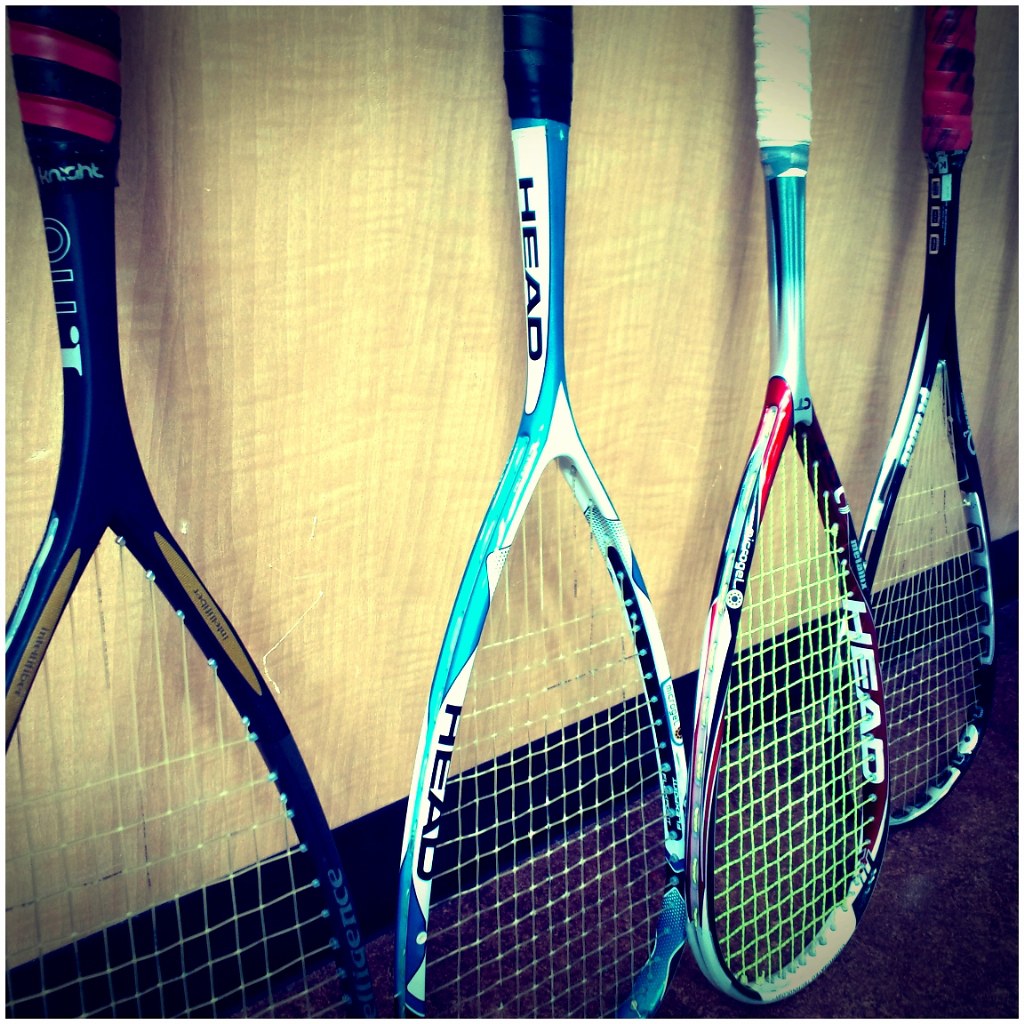This photograph showcases four racquetball racquets hanging diagonally on a light tan wooden wall with a chocolate brown or black border at the bottom. Due to the perspective, the racquets appear to decrease in size from left to right. Each racquet features the brand name "HEAD" in either white or black lettering on the frame. The racquet on the far left has a black frame and handle with diagonal red lines at the base. Next to it, there's a blue and white racquet with a black taped handle. The third racquet has a multi-colored frame in shades of blue, black, red, and white, with a white handle wrapping. The one on the far right is primarily black and white with a red taped handle. The racquets are leaning upright against the wall, resting on their frames, giving a dynamic and professional appearance.